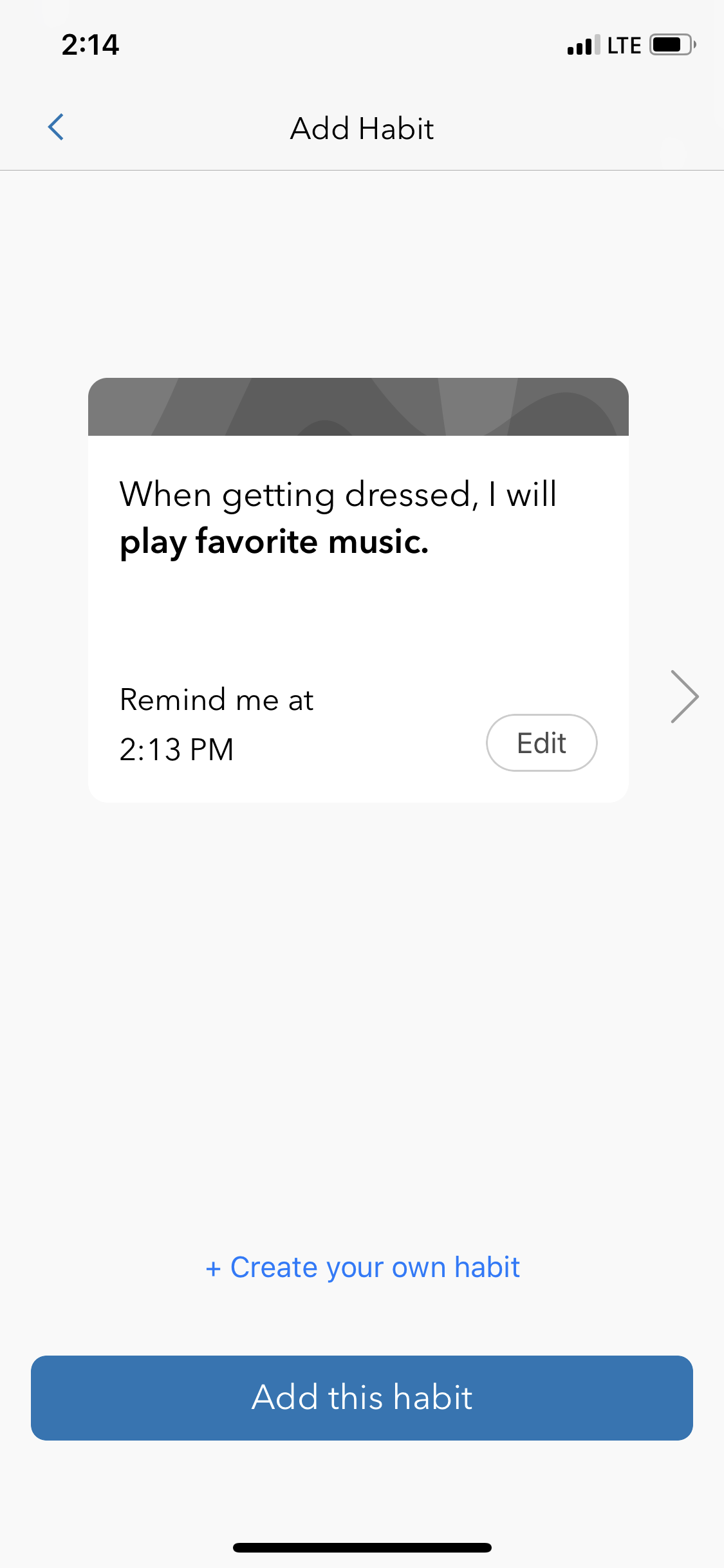The image is a vertically rectangular screenshot from a cell phone app, displaying a habit-tracking interface. The background is a light gray color. 

At the top left corner, the time is shown in black (2:14). On the top right, there are several icons: the cell signal bar, LTE designation, and the battery level icon. 

Beneath these icons, on the left, there is a blue back arrow. Centrally placed, in black, is the title "Add Habit". 

In the middle of the frame, there is a central window display with the text: "When getting dressed, I will play favorite music. Remind me at 2:13 p.m." At the bottom right corner of this display, there is an edit button.

Further down, near the bottom of the image, there is a plus symbol followed by the text "Create Your Own Habit". Directly beneath it is a blue button with white text reading "Add This Habit". 

At the very bottom of the screenshot, there's a black horizontal bar that does not extend the full width of the frame but is centered just above the bottom edge.